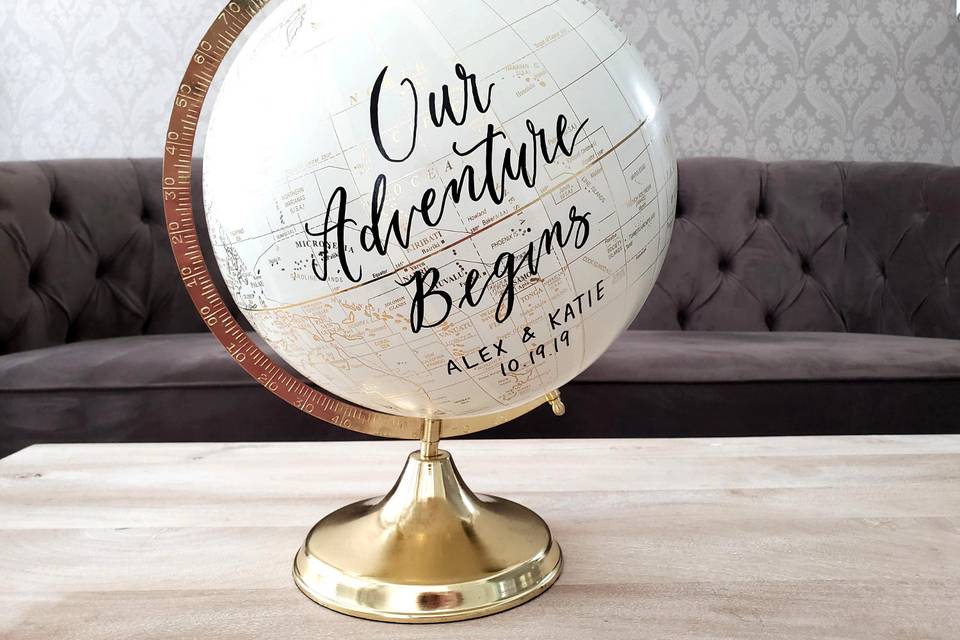The image features a small, intricately designed white globe with light tan and gray continents, used as a wedding memento. Bold cursive letters across the globe read "Our Adventure Begins," with "Alex and Katie" followed by the date "10.19.19" printed below in capital letters. The globe is detailed with a thin gold line at the equator and is mounted on a gold base. It sits about three-fourths of the way down on a light brown, stained wooden table. The backdrop includes a long tufted gray couch set against grayish wallpaper with an intricate design, reminiscent of lions' manes, adding to the elegant atmosphere.